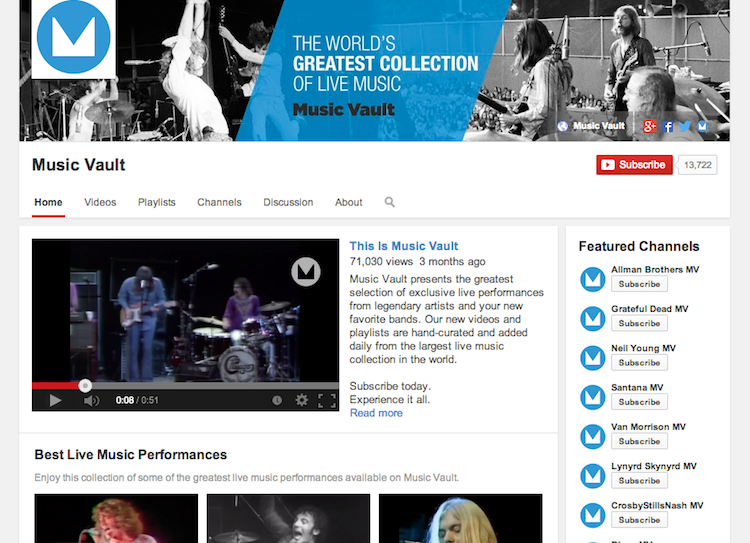The image displays a screenshot of a YouTube channel named "Music Vault." At the top, the channel banner showcases a series of photos from various concerts, with the text "The world's greatest collection of live music, Music Vault" prominently displayed in the center. To the right of the banner is the red "Subscribe" button, and at the time of the screenshot, the channel boasts 13,722 subscribers.

Below the banner are navigation tabs labeled Home, Videos, Playlists, Channels, Discussion, About, and a Search bar, providing easy access to different sections of the channel. The featured, or pinned, video titled "This is Music Vault" sits prominently on the page, having garnered 71,030 views and posted three months prior to this screenshot. The video's description reads: "Music Vault presents the greatest selection of exclusive live performances from legendary artists and your new favorite bands. Our new videos and playlists are hand-curated and added daily from the largest live music collection in the world. Subscribe today. Experience it all."

On the right sidebar, there's a section titled "Featured Channels," highlighting other channels associated with Music Vault. The detailed layout and strategic placement of elements reflect a well-organized and inviting channel geared towards music enthusiasts.